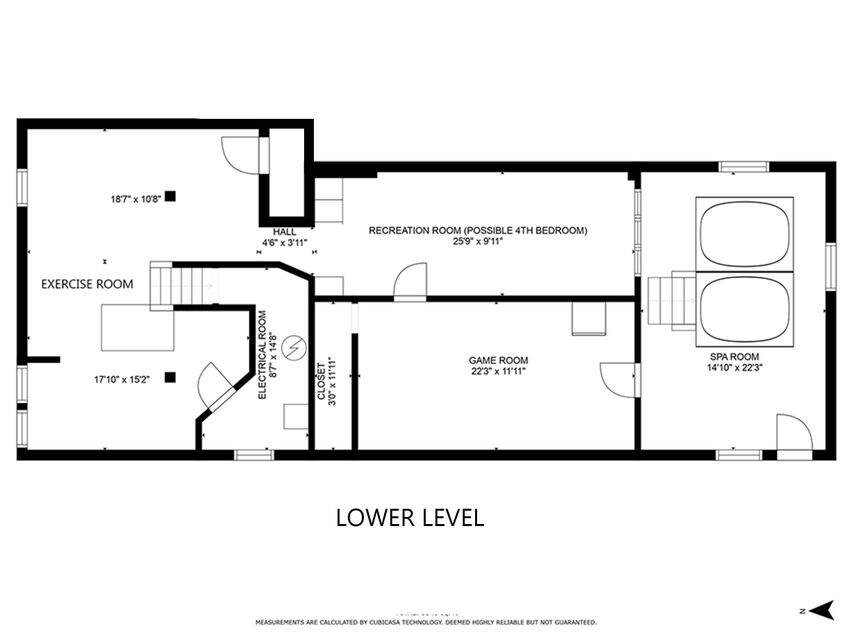A detailed schematic drawing of the lower level of a building is shown. The exterior walls and main hallway are represented by thick black lines, while interior walls are indicated by thinner black lines. Various rooms are labeled with their dimensions. The lower level features an exercise room, a recreation room, and a potential fourth bedroom. Each room is indicated with precise measurements.

The schematic also includes a hallway, an electrical room, and utility symbols such as a circle and a box, likely representing the HVAC unit and hot water heater, respectively. Doors, steps, and windows are depicted, though the windows are not specifically marked. 

A game room with a closet, as well as a spa room featuring a rectangle with two ovals, presumably indicating a hot tub, are illustrated. There is another hot tub, with access via steps, and this area appears to have the only exterior door on this level.

Additionally, a north marker is present to provide orientation. Despite some elements not being labeled, the schematic thoroughly outlines the lower level's layout, giving a comprehensive view of its structure and functionalities.